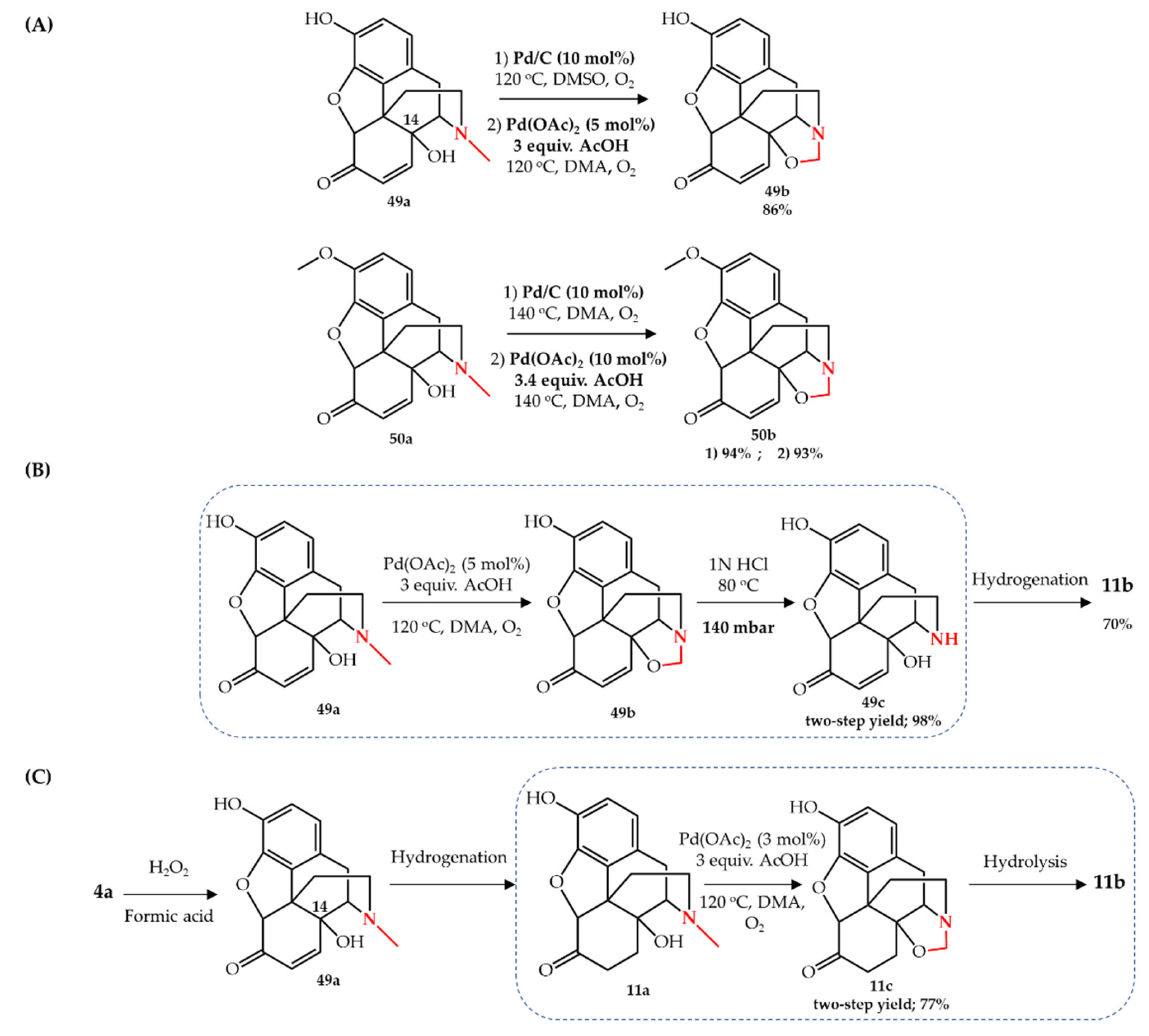The image depicts a detailed scientific schematic of molecular drawings and chemical reactions. 

**Section A:**
- **Step 1:** This step involves the chemical notation "1. Pd/C (10 mol%) 120°C, DMSO, O₂," followed by an arrow pointing to the right.
- **Step 2:** The next notation is "Pd(OAc)₂ (5 mol%), 3 equiv. AcOH, 120°C, DMA, O₂," also with an arrow to the right. Corresponding molecular structures are illustrated alongside these descriptions.

**Section B:**
- This section focuses on hydrogenation, indicating "70% yield," followed by relevant molecular drawings.

**Section C:**
- Mentions formic acid as a reagent, with an arrow leading to "hydrogenation."

Below each segment, additional molecular drawings and notation are present, including hydrolysis labeled as "11B".

Overall, the image captures a sequence of chemical reactions, each accompanied by precise details such as concentrations, temperatures, and conditions, illustrated with corresponding molecular structures.